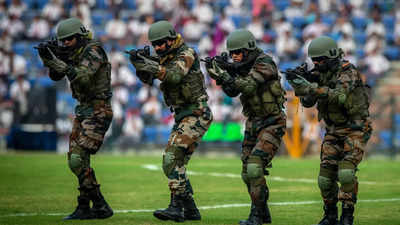This vividly detailed color photograph captures an outdoor scene on what appears to be a sports or athletic field, recognizable by the green astroturf and lined markings. In the background, a blurred crowd fills the stadium stands, intently watching the spectacle unfolding before them. The focal point of the image is four military personnel, presumably men, dressed in full camouflage gear. Each soldier is outfitted with black boots, green helmets, bulletproof vests, and black sunglasses. They are also equipped with backpacks and scarves that leave only their faces exposed. The men are walking in a line with knees slightly bent and bodies hunched forward, their expressions stern and focused. Cradling black automatic rifles, the soldiers hold their weapons in a ready-to-fire position, aimed ahead as they move. This poised and intense formation suggests they are part of a choreographed display or demonstration, perhaps during a special event or show at the stadium.